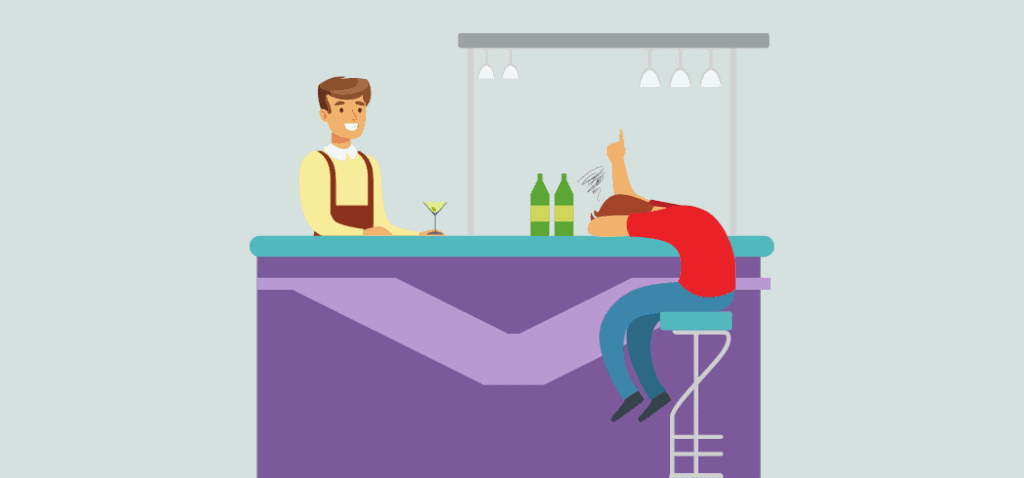In this computer-generated illustration, a cartoon-like bartender is preparing to serve a drink to a seemingly drunk patron at the bar. The bartender, positioned on the left, is adorned in a burgundy apron, a yellow long-sleeve shirt, and has reddish-brown hair coupled with a smile. He stands behind a bar with a blue and purple hue, reaching out with a wine glass containing a pale golden or light green beverage.

Overhead, five lights hang—two on the left and three on the right—illuminating the scene. The patron, situated on the right, is slouched over the bar, appearing disoriented with action lines signifying confusion above his head. He sports a red shirt and jeans, and brown hair that matches the bartender's. In front of him lie two bottles, one green with a gold label. The bar itself features a light purple chevron pattern underneath. Both characters are highly animated, resembling emojis or cartoon figures, adding a playful, whimsical feel to the scene.